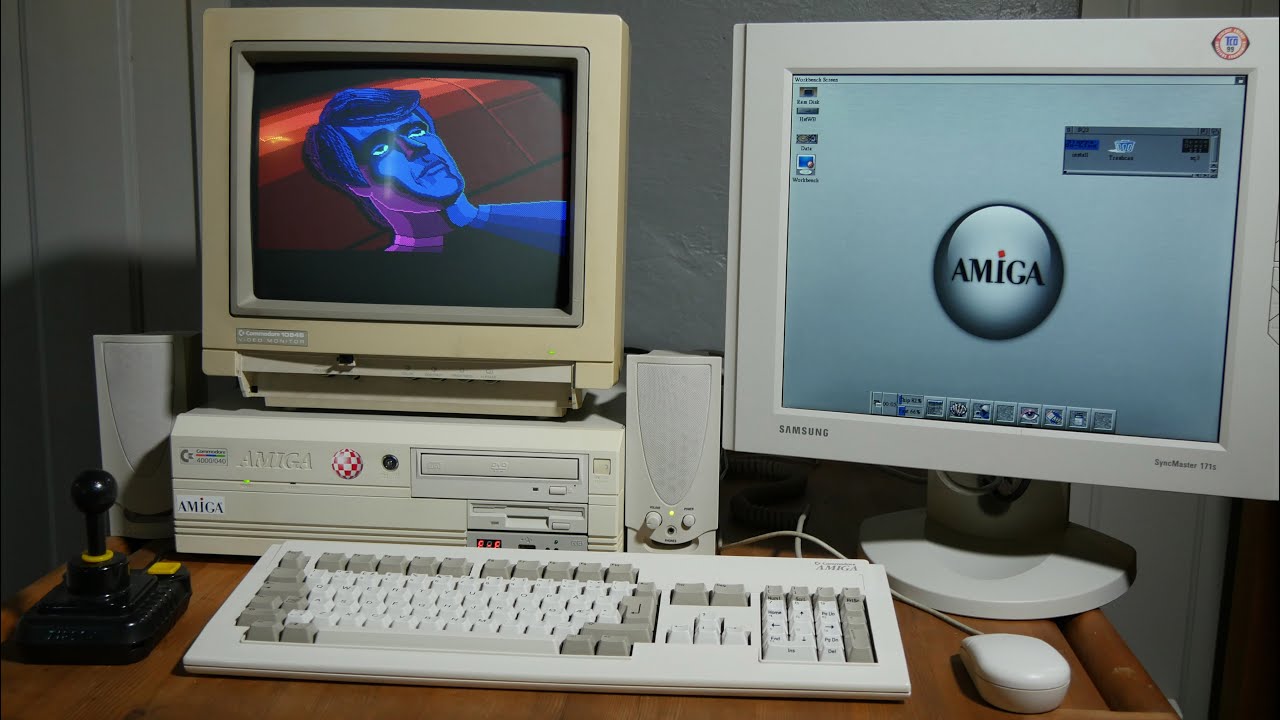The indoor photograph showcases a vintage computer setup with two distinct monitors. On the left is an old-style, yellowed-gray CRT monitor displaying a detailed illustration of an animated man, purple in color, lying on a red background. The monitor rests on a computer tower labeled "Amiga." To the right, a second screen, light gray in color and branded with the Amiga logo (featuring a red dot over the 'I'), exhibits a web interface. The desk beneath is brown and holds a white and gray keyboard, a matching white mouse, and a black joystick to the keyboard's left. This entire setup is surrounded by additional small speakers. The room features white walls with a door on the left side of the image, enhancing the nostalgic atmosphere of this vintage workstation.